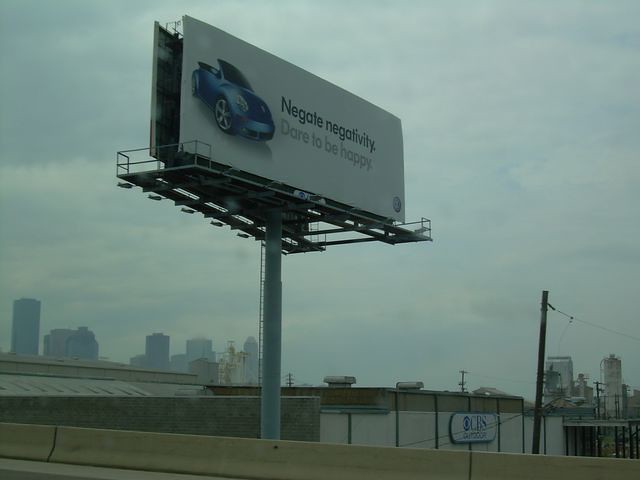This image features a vivid scene that initially appears to be a photograph of a billboard in a bustling city. Upon closer inspection, however, the scene has a slightly surreal, almost too flawless quality that suggests it might be a still from a video game. The focal point of the image is a prominent billboard viewed from the side, as though the viewer is standing on the road and looking up past a cement divider.

The billboard's message, "Negate Negativity, Dare to Be Happy," is emblazoned in bold letters next to an image of a sleek blue convertible sports car. A small round logo in the bottom right corner hints at it being a BMW advertisement. The billboard itself is mounted on a sturdy metal post, standing tall amidst a commercial area.

In the background, a building features a placard, possibly indicating it is a store or some form of facility. Further adding to the urban environment are a telephone pole or power pole and several skyscrapers that pierce the hazy sky, contributing to the scene's cityscape. This blend of detailed urban elements and the dreamy, almost perfect quality of the image makes it both familiar and intriguingly otherworldly.